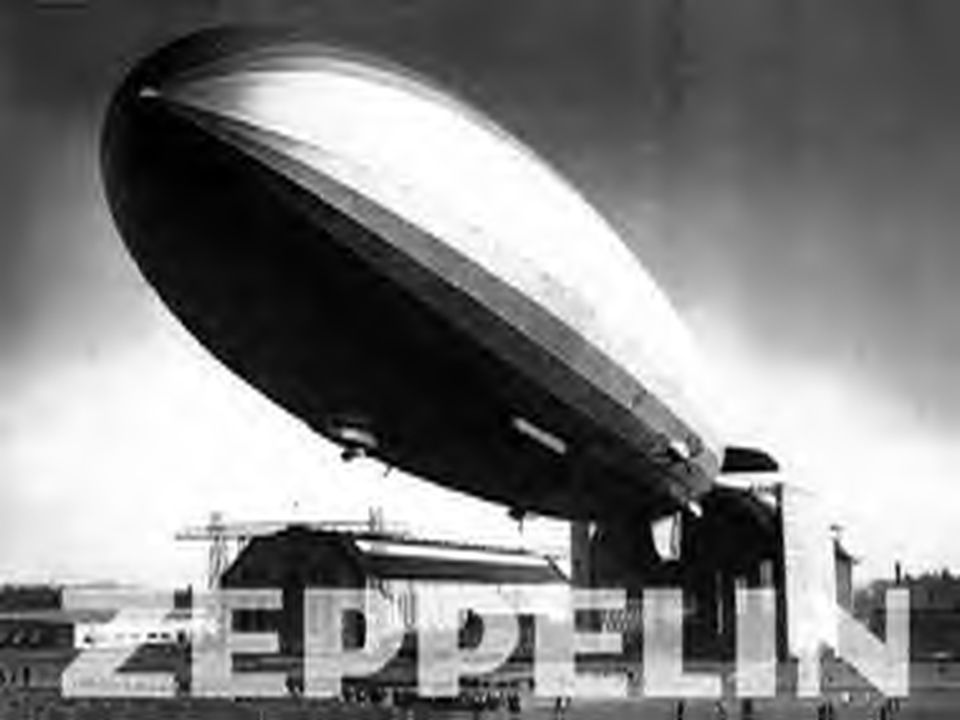This is an old, black and white photo, slightly blurry and worn with age. In the center, prominently pointed towards the upper left corner, is a large Zeppelin, which appears black on the bottom and whitish-gray on the sides, resembling a massive bullet. The background reveals a cloudy sky varying in shades of black, gray, and white, transitioning from dark at the top to lighter tones in the middle and bottom sections of the image. Below the Zeppelin, in large, all-cap white letters, reads "ZEPPELIN," centered at the bottom of the photo. On the ground, diminutive and indistinct figures, likely people, and some buildings are visible, though they are small and somewhat obscured by the photo's blurriness. The scene is outdoors, and the ground level details, alongside the cloudy sky, evoke a historical atmosphere.